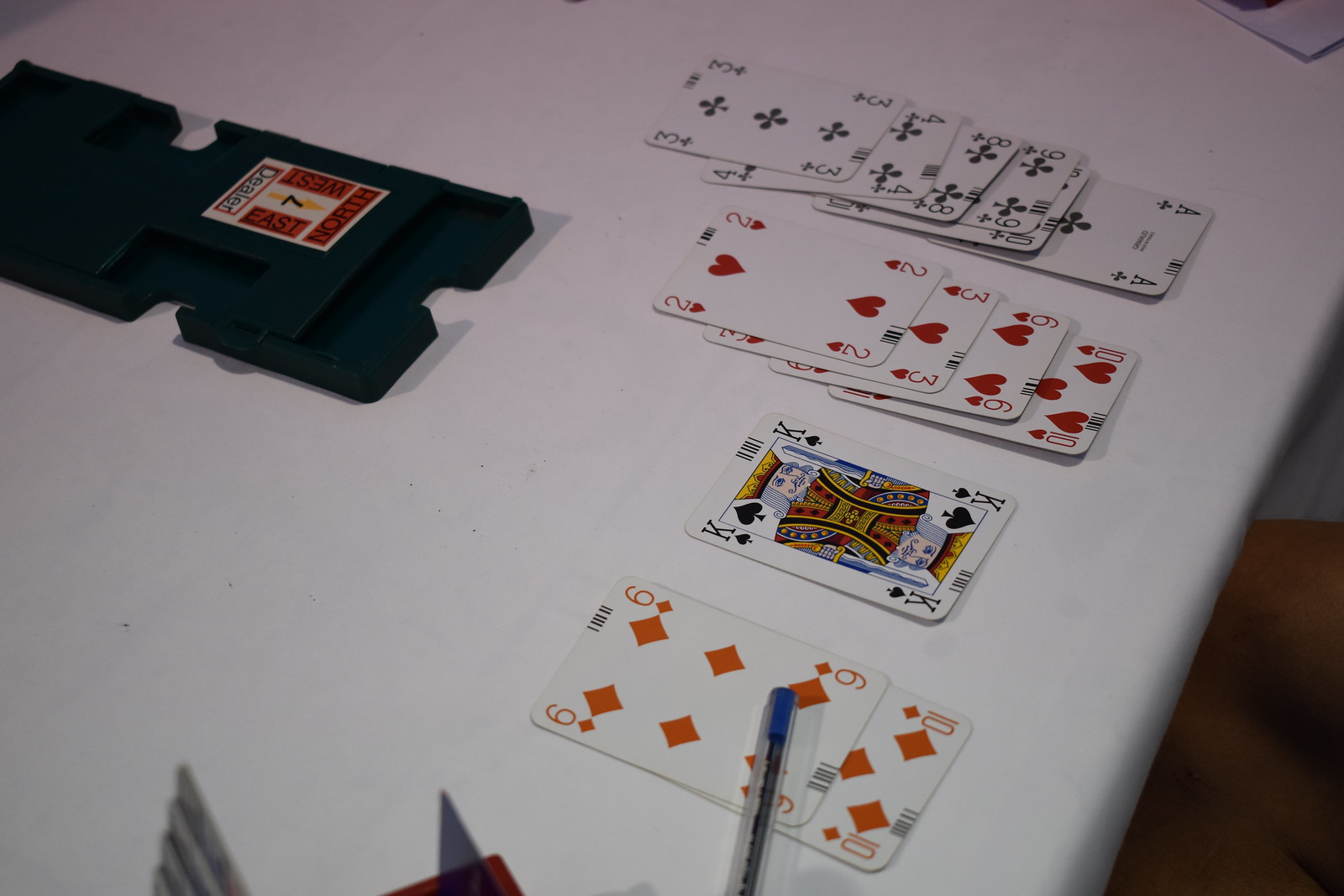The photograph highlights a large white table where someone is engaged in a card game, potentially solitaire. In the upper left-hand corner, there is a black rectangular device with a sticker labeled '7' and the word 'Dealer', suggesting it is some sort of card dealing apparatus. 

At the lower section of the table, arranged from bottom to top, are two red cards: the 6 of diamonds and the 10 of diamonds, accompanied by a blue ink pen placed on top. Moving rightward from these, the black king of spades is positioned. Above it, a sequence of four red heart suit cards is neatly stacked: the 2 of hearts, the 3 of hearts, the 6 of hearts, and the 10 of hearts.

Further to the right, another set of cards progresses vertically, consisting of the 3 of clubs, 4 of clubs, 8 of clubs, 9 of clubs, 10 of clubs, and concluding with the ace of clubs at the very bottom. In the lower right-hand corner of the image, part of a person's limbs—either arms or legs—are faintly visible, adding a human element to the scene.